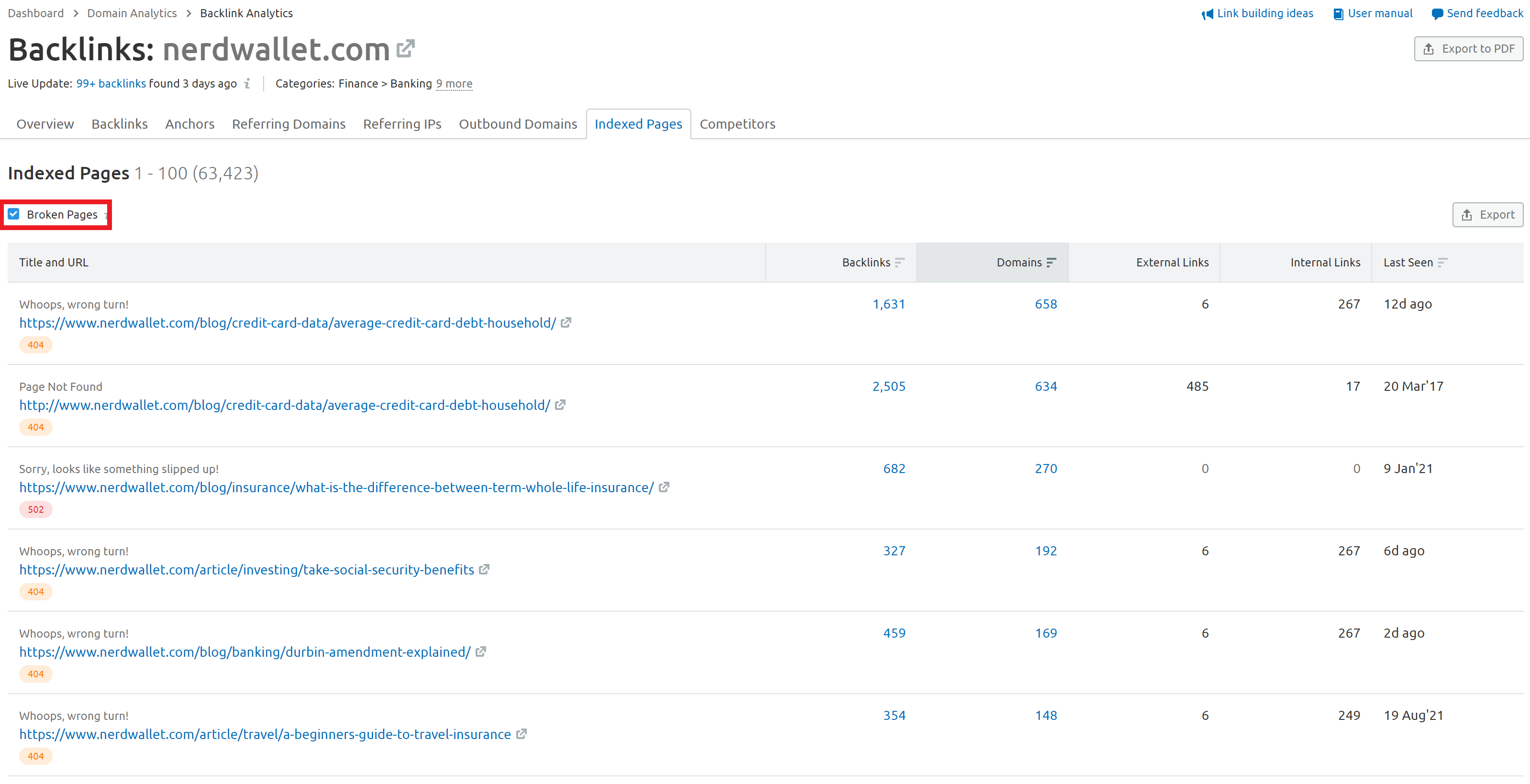**Detailed Caption:**

The image features a screenshot of a web-based dashboard, which is formatted in a landscape layout. The dashboard's background is predominantly white. In the top-left corner, small, barely legible text likely indicates the specific section of the website being viewed. Directly below this small text, "backlinks: nerdwallet.com" is written in bold, next to an icon that allows users to navigate to nerdwallet.com.

On the upper right side of the dashboard, there are three clickable blue text sections, with a small gray button situated underneath them. Beneath this header area, a navigation bar with eight tabs stretches horizontally across the dashboard. The penultimate tab is selected, indicated by its blue color and an encasing gray outline.

Below the navigation bar, on the left side, "index pages" is prominently displayed in bold. Next to it, in regular font, it states "1-100 (63,423)", suggesting a pagination format with a total count of 63,423 indexed pages.

The main body of the dashboard comprises a data table, with six columns arranged horizontally. The first column is the longest and lists URLs along with some associated text. Each entry in this column includes a small, unreadable button at the bottom. The subsequent columns have titles at the top and display corresponding data as numbers down the rows, except for the last column, which seems to contain date entries or an indication of how many days ago the data was relevant. Each row in the table starts with an entry in the first column and is followed by data in the subsequent columns. There are a total of six visible rows in the table.